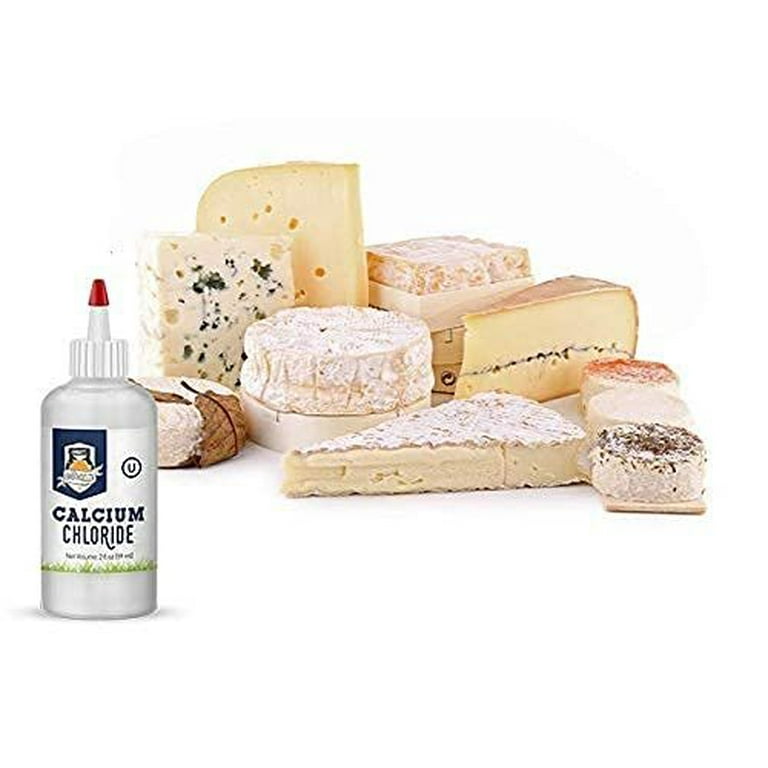This vivid photograph showcases an assortment of around ten distinct types of cheeses and baked goods, artfully arranged as if displayed in a deli. The cheeses vary in texture and appearance, predominantly pale yellow or white, with some topped with a powdery substance resembling powdered sugar. Among the assortment are cheeses that intriguingly resemble Little Debbie or Hostess Ding Dongs, adding a whimsical touch. Some cheeses feature colorful toppings; one has a green topping, another is brown, and a third displays a striking red top. A bottle of calcium chloride, prominent on the left side with its white and grey hues, a red cap, and a blue logo with grass imagery, introduces an unexpected element to the scene, hinting at its possible use in cheese production. The background is stark white, further highlighting the detailed textures and hues of the cheeses and baked goods.